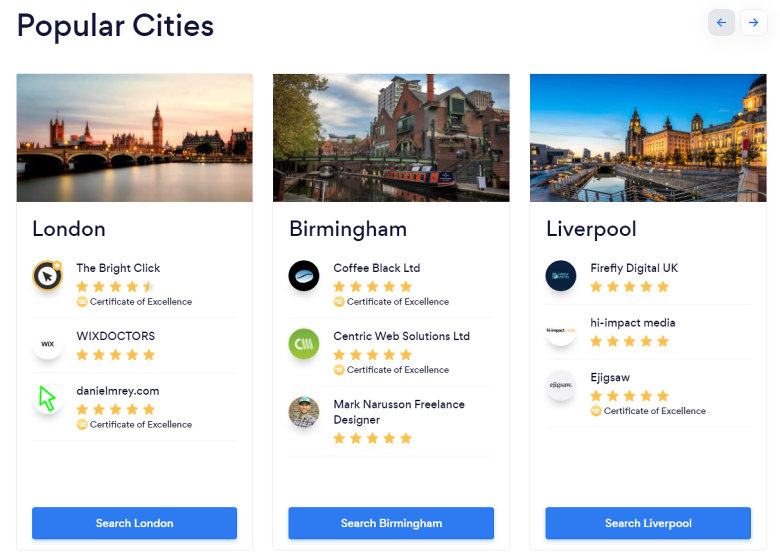At the top left, the text "Popular Cities" is displayed in a bold black rounded font, resembling Century Gothic. To the right, there are two small rounded squares, each containing a blue arrow. The left arrow, set against a light gray background, points left, while the right arrow, set against a white background, points right.

The first highlighted image showcases London, featuring the iconic London Bridge. The sky transitions from light blue in the top left to a pink hue in the center, complemented by white clouds in the top right. Below the image, "London" is written in a dark gray bolded font on a white background. Next to the text is a circular icon with a black border and a black mouse pointer pointing to the upper left. This icon is surrounded by a yellow outer border and a yellow circle to the right. Adjacent to the icon, the text "The Bright Click" appears in black font, followed by a rating of four and a half out of five stars, with four and a half stars filled in orange and the remaining half star in light gray. Additionally, there is an orange circular icon with a 'C' and the phrase "Certificate of Excellence" in black.

The second image depicts Birmingham, featuring a brown or red brick building and a sky filled with wispy clouds. An oak tree stands to the left, and a red train is visible in the bottom right corner. Below this image, "Birmingham" is written in black lettering. Accompanying this text is a black rounded icon depicting a coffee bean with a gradient from dark blue at the top to light blue at the bottom. To the right of the icon, the text "Coffee Black LTD" appears, followed by a perfect rating of five out of five stars. A similar "Certificate of Excellence" icon as seen in the London section is also present.

The third image features Liverpool under a bright blue sky. Below this image, "Liverpool" is written in black font, completing the visual representation of these popular cities.